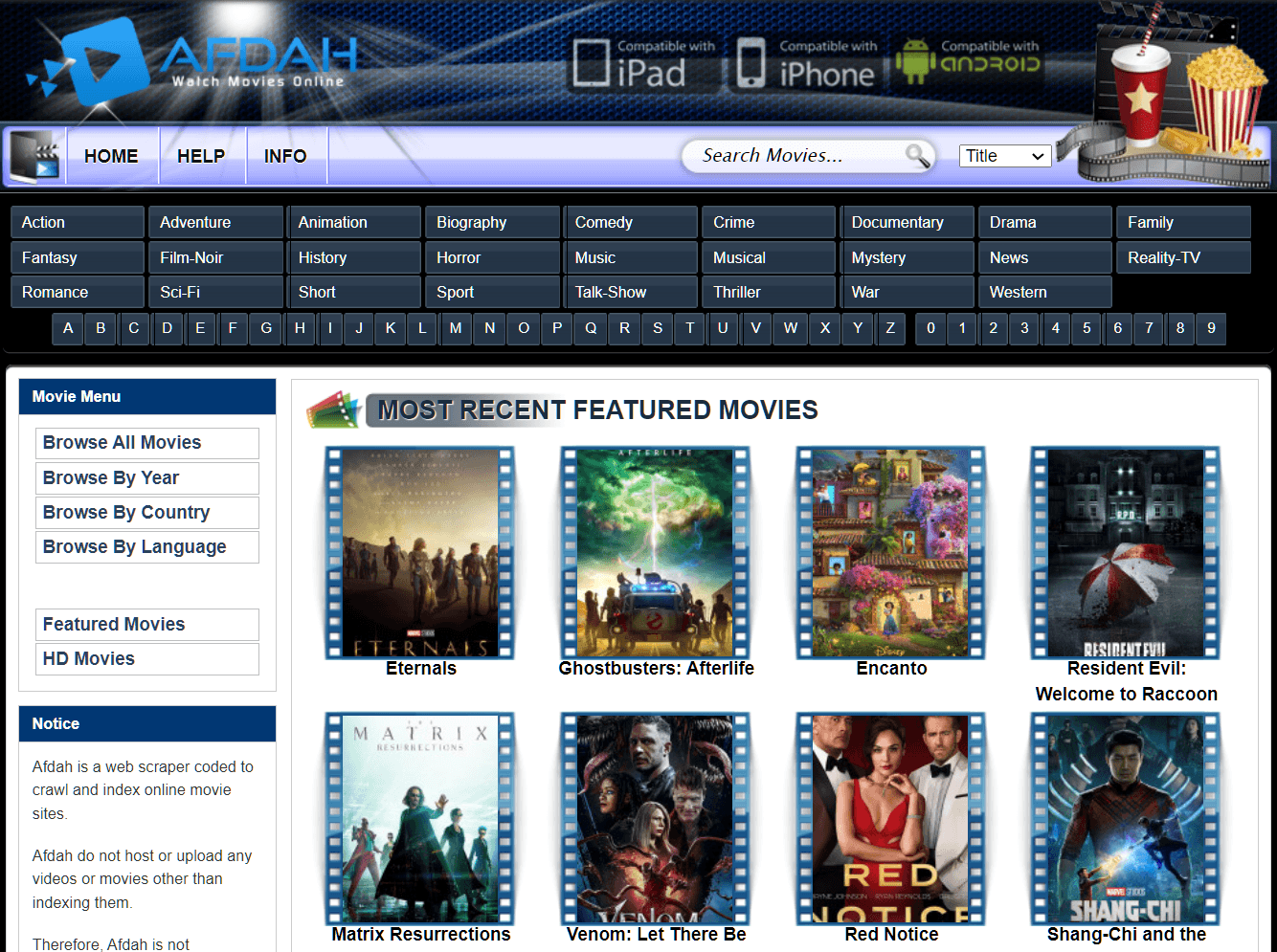The AFDA website, prominently titled "Watch Movies Online," features a distinctive blue logo resembling a YouTube play button on the far left of its header. The header's background is adorned with a stylish light stream graphic. Directly below the logo, AFDA is written, followed by the tagline "Watch Movies Online" in white text.

On the left side of the header, a small text box highlights device compatibility with images and labels for iPad, iPhone, and Android. In the top right corner, an illustration shows a drink, movie popcorn, and a film reel, emphasizing the site's entertainment focus.

The light blue navigation bar beneath the header offers quick access to "Home" and "Help/Info" sections, accompanied by a search bar where users can find movies by title or genre. The expanded genre section below is marked by dark blue text detailing various genres. An alphabet and number section are also present for browsing.

The main section of the page currently displays "Most Recent Featured Movies," focusing user attention on the latest additions. To the left, a sidebar labeled "Movie Menu" provides options to browse all movies, filter by year, country, language, and access featured and HD movies. An "In Notice" section is listed underneath the menu for important updates or announcements.